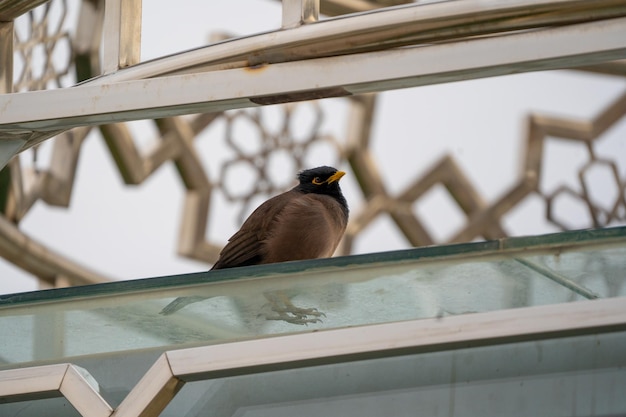In a photograph taken outdoors on a bright, sunny day, the focal point is a plump bird perched on a clear glass surface, which could be plexiglass or heavy glass. The bird is notable for its brown chest and feathered body, with its head featuring darker feathers—appearing almost black. It has a gold beak and yellow markings around its eyes. Its small bird feet are firmly planted on the glass. The background reveals a structure with gold and rusting metal elements, including a rod and ornate filigree work consisting of hexagons with circles inside them. A gold bar runs from the bottom left to the right part of the photo, with another metal piece spanning across. The sky in the backdrop appears clear and white, providing a soft contrast to the intricate metalwork and the bird's detailed features. The bird, looking to its right with its beak slightly raised toward the air, creates a calm yet observant scene.